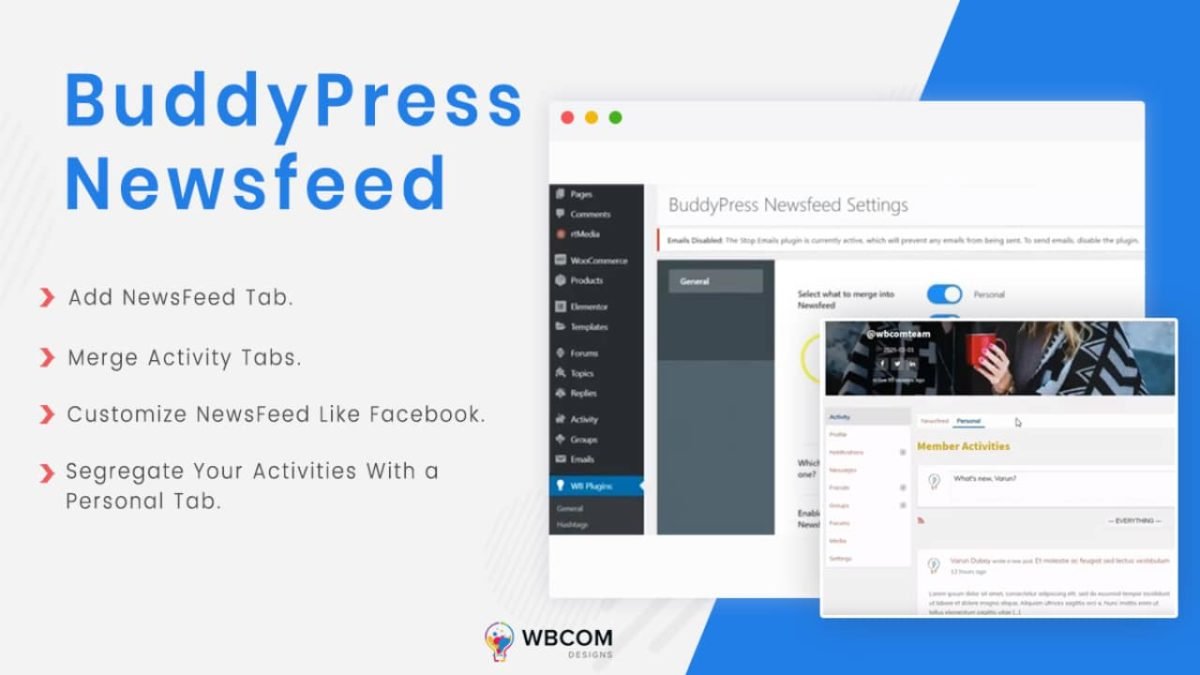Screenshot of a website displaying the BuddyPress News Feed settings page. The background transitions from a very light gray on the left to a medium royal blue at a 30-degree downward angle as it approaches the right side. 

On the left side, large uppercase letters spell out "Buddy Press News Feed." Below this title, there are four red arrows pointing to the right, each followed by black text in a grayish font. The text next to the arrows reads as follows:
1. Add News Feed Tab
2. Merge Activity Tabs
3. Customize News Feed Like Facebook
4. Segregate Your Activities with a Personal Tab

At the bottom center of the image, a colorful light bulb icon is visible. To the right of the light bulb, bold black letters spell out "WBCOM," with the word "Designs" in small block letters underneath.

On the right side of the image are several web page previews. One full web page has a gray border and a white background, featuring a black vertical tab with symbols indicating various actions. A blue-highlighted section labeled "Edit Pages" contains a gray bar with options to toggle features on and off. This section represents the BuddyPress News Feed Settings.

Further down on the right side, a smaller web page is open, with a banner at the top showing a hand holding a mug of coffee alongside clothing items. This page is titled "Member Activities" and features activity bars and feeds, providing a model for customizing the user's page.